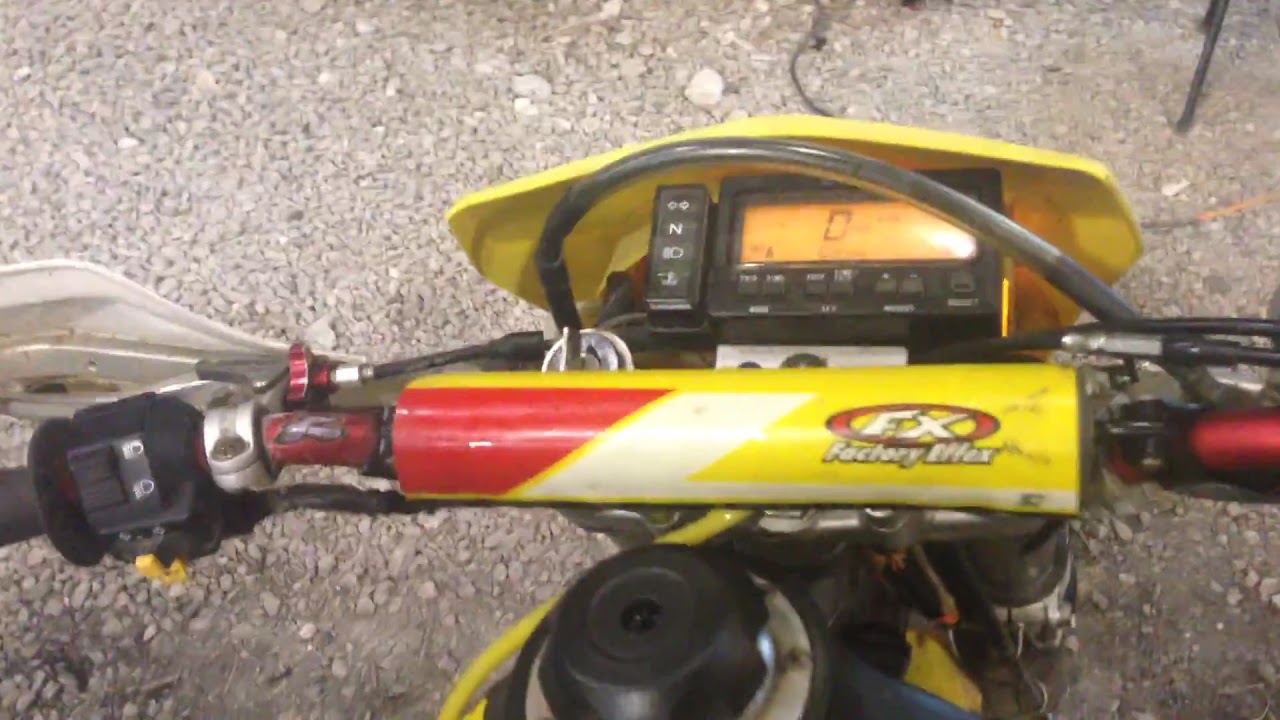The image captures a top-down view of what appears to be an electric or motorbike, set against a gray, gravel-covered ground. Central to the composition are the brightly colored handlebars, featuring a mix of yellow, red, black, and white. Above the handlebars, a black horizontal rectangular digital display with an orange screen shows a black zero, surrounded by buttons with white text. Additional details include a black tube arching from the right handlebar towards the left, looping over the display. To the left, there is a yellow shield, possibly covering a motor component, marked with "FX." The bike is equipped with a gear shifter, light switch, and vertical buttons with icons related to lights and gear positions. The foreground prominently features elements of the bike’s body and possibly part of the engine or motor, adding to the complexity and utility of the vehicle.